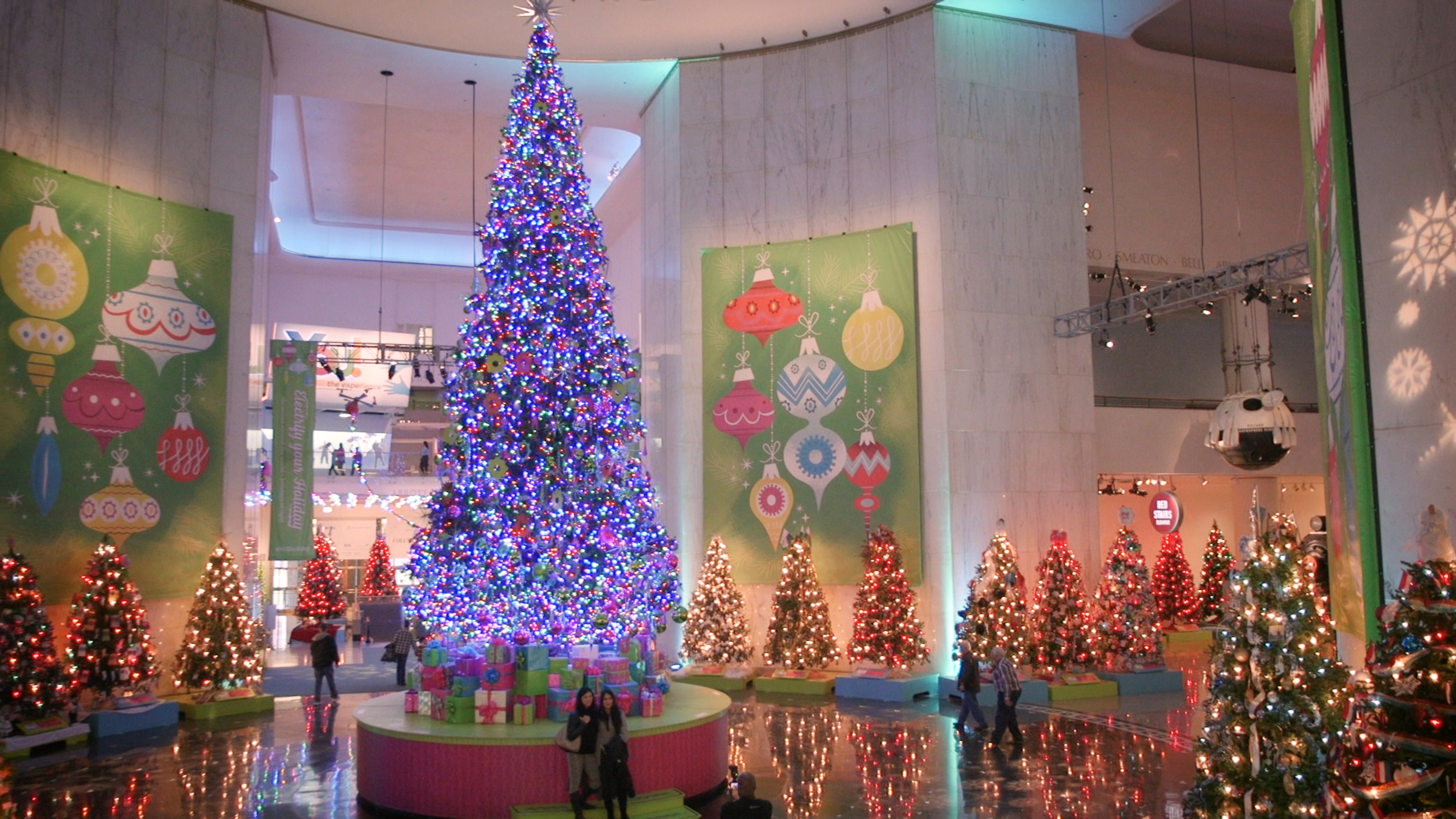The image depicts a festive atrium of what appears to be a theater or a mall, characterized by its towering ceilings that soar approximately 20 to 30 feet high. The main focal point is a colossal Christmas tree, adorned with a dazzling array of purple, pink, lavender, and blue lights, which stretches up to the high ceiling and sits prominently on a round pedestal with hues of blue, pink, and green. Beneath this central tree, numerous Christmas presents are neatly arranged. Two dark-haired women are posing for a photograph, with a man holding a camera in front of them.

Surrounding the central tree, the space is filled with several smaller Christmas trees, all intricately decorated with mainly yellow and red lights, alongside a mix of yellow and green ones. The ambiance is enhanced by Christmas murals and large paintings of Christmas ornaments embellishing the walls. The layout of the building reveals two additional levels where people can be seen against the balconies, watching the festive scene below. The atrium is bustling with visitors walking around, absorbing the joyous holiday atmosphere.